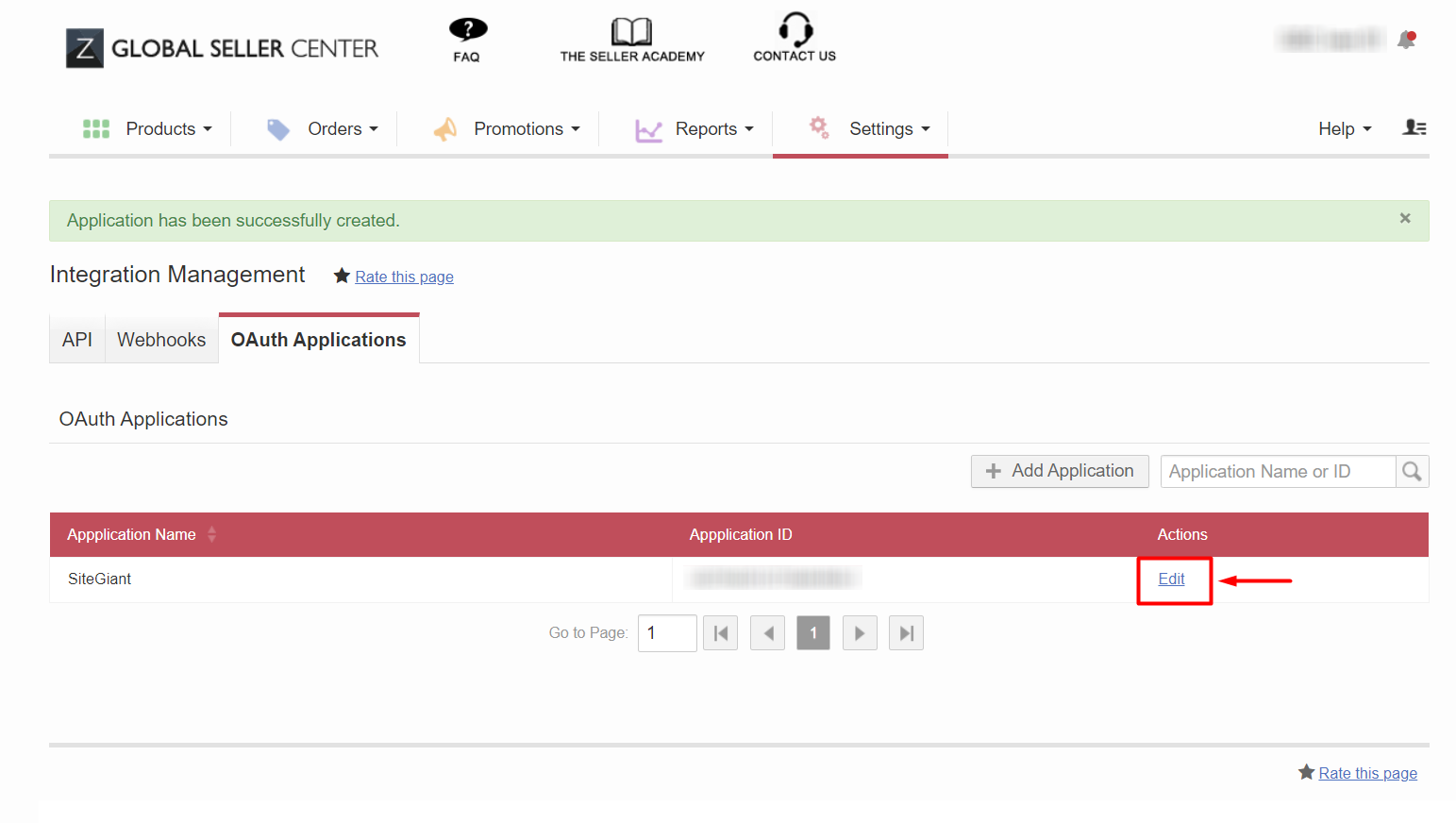The image depicts a digital interface, prominently featuring a logo comprising the letter "Z" in white within a black square. Next to the logo, bold black letters spell out "Global Seller Center." Adjacent to this text is a black circle with a question mark inside, labeled "FAQ."

Below the logo and FAQ section, there's an open book icon accompanied by the text "Seller Academy." Following this is an illustration of a headset with a microphone, next to which reads "Contact Us." The user's name is redacted in this section.

At the top of the interface, a navigation menu displays several options: "Products," "Orders," "Promotions," "Reports," and "Settings," each with a drop-down arrow. The "Settings" option is highlighted in pink and features a gear icon. On the opposite side of this menu, there's a "Help" section.

Beneath the main navigation, a green notification bar announces that an application has been successfully created, with an option to close this message marked by an "X." Below this notification, text indicating "Integration Management" is displayed. A highlighted blue option labeled "Rate This Page" is present, alongside another highlighted section titled "OAuth Applications."